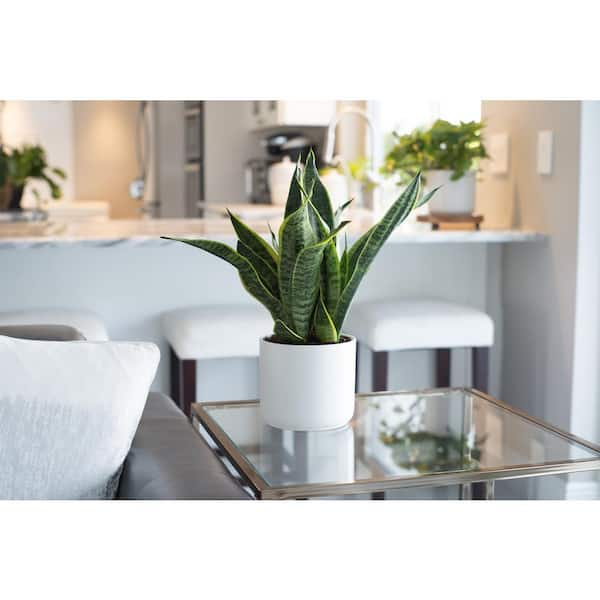This high-quality photograph captures a sophisticated corner of a living room, displaying a minimalist aesthetic dominated by white and neutral tones. The focal point is a small snake plant with tall, green leaves featuring lighter green edges and subtle horizontal stripes, nestled in a pristine white pot. This plant sits on a sleek, square glass end table with a metallic rim, accentuating the modern design elements of the space.

Adjacent to the table is a brownish-gray sofa adorned with a white pillow, adding a touch of comfort and contrast. In the background, a white bar with three white-cushioned barstools is visible, further emphasizing the room's color palette. Atop the bar is a blurred glimpse of another houseplant in a white pot, maintaining the room's cohesive decor. Beyond the bar is a kitchen area featuring a window, a sink, and what appears to be a coffee pot. The setting exudes an air of affluence and simplicity, highlighted by the understated yet elegant choice of furnishings and decor.